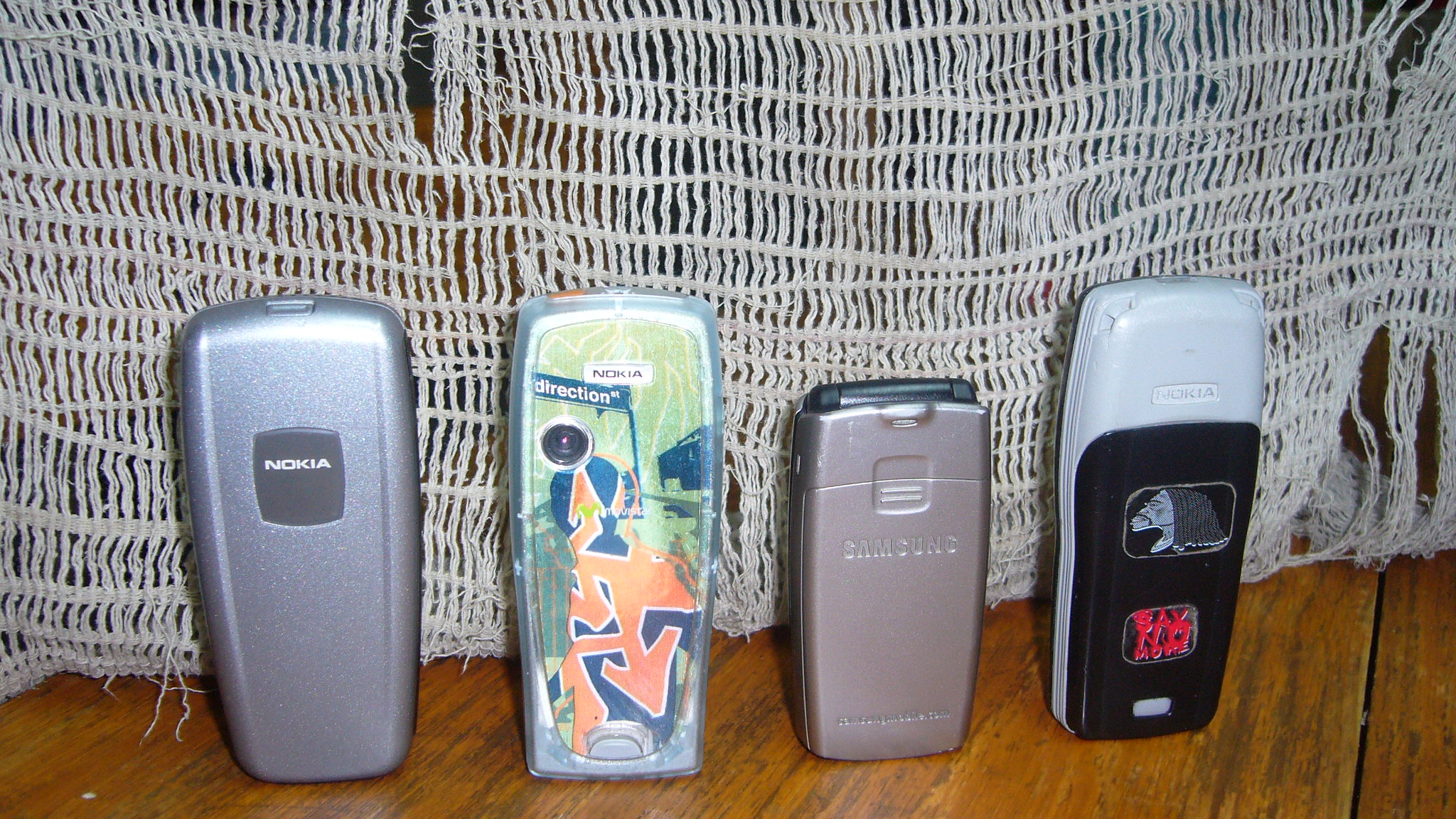A detailed photograph shows four old mobile phones lined up on a brown wooden floor against a white string background, possibly near a couch or covered table. On the left, there's a sleek, shiny silver Nokia phone with a metallic cover, resembling the texture of a football lid, featuring a camera on the top left. Next to it is a Samsung flip phone with engraved writing on its gray surface. The third phone from the left has a greenish-gray background with a distinctive red symbol in the middle, flanked by black accents. The final phone on the right, a Nokia, is characterized by its white upper part and black bottom with some red details. All the phones vary in color and size, with the smallest being the flip phone, and they showcase a range of designs from retro to more contemporary styling.